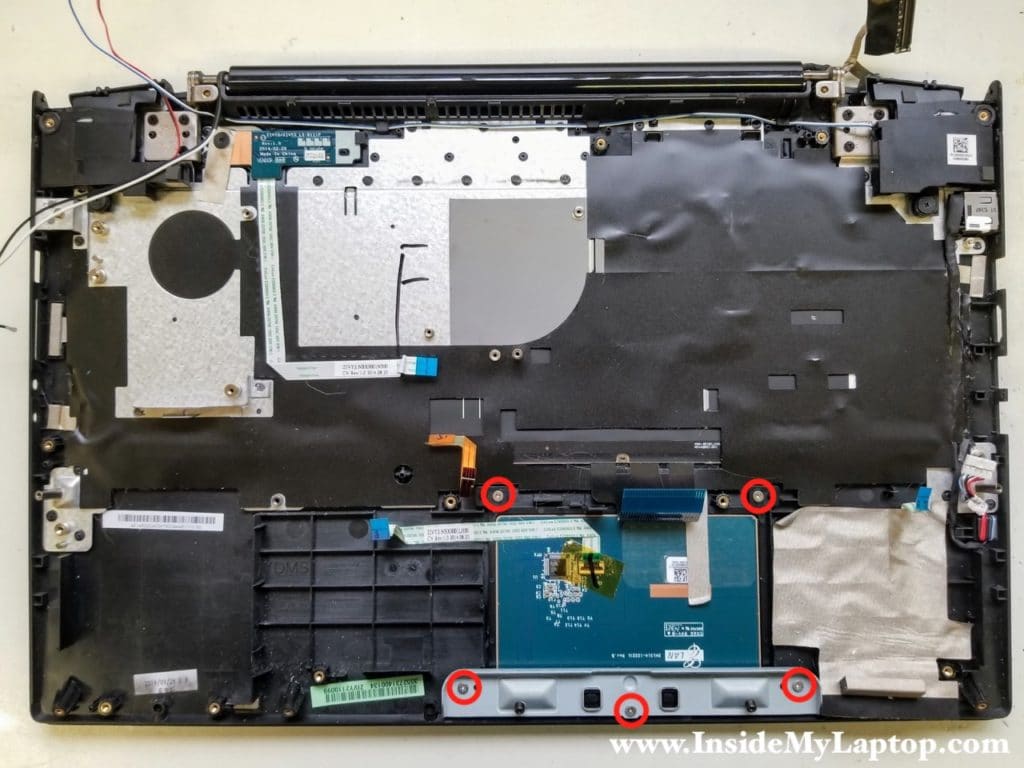This image showcases the bottom of a disassembled laptop with its cover removed, exposing its intricate internal components. Predominantly black with chrome details, the laptop's insides reveal a variety of other colors, including green, blue, red, teal, tan, and orange, contributing to a complex and detailed visual. Highlighting the key screws for removal, five red circles are meticulously drawn near the bottom. In the top left corner, there are wires in red, blue, black, and white, exemplifying the meticulous internal wiring. The top right features a white label with a QR code, and in the bottom right, a piece of paper with a blue tab is slightly covering another component. Centrally, a blue circuit board adorned with a piece of yellow tape contrasts against a black section covered in a specific material, with a green sticker positioned slightly to the left. The entirety of the laptop rests on an off-white table, taking up the entire image, with the website www.insidemylaptop.com printed in white at the bottom, offering a technical glimpse into the device’s inner workings amidst an off-white background likely in someone's computer room.